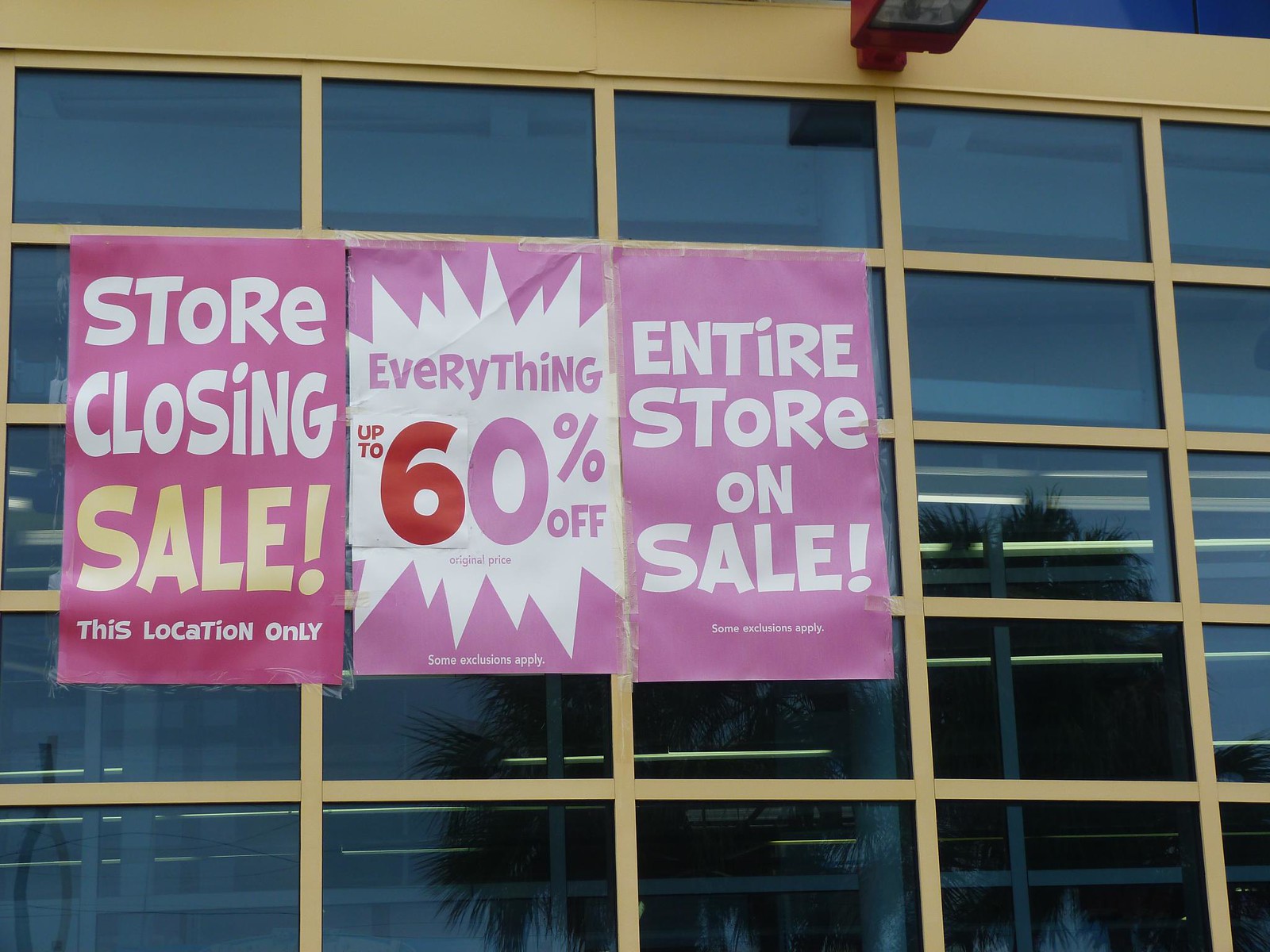The image depicts a storefront window announcing a store closing sale. Three prominent signs are displayed in the window, positioned left, middle, and right. The text details are as follows:

1. The top of the image features gold-colored text proclaiming the store closing sale, which is clearly limited to this location only.
2. The phrase "Store Closing Sale" is rendered in bold yellow text.
3. On the left side of the image, white text reads "This location only."
4. The background is a vibrant mix of pink and red hues, creating an eye-catching contrast.
5. White text on the upper left also states "Some exclusions apply."
6. Central to the image, a larger sign announces "Everything up to 60% off" in striking white and pink text.

The signage collectively emphasizes the urgency and scope of the sale within this specific store, set against a visually appealing background designed to draw customers' attention.